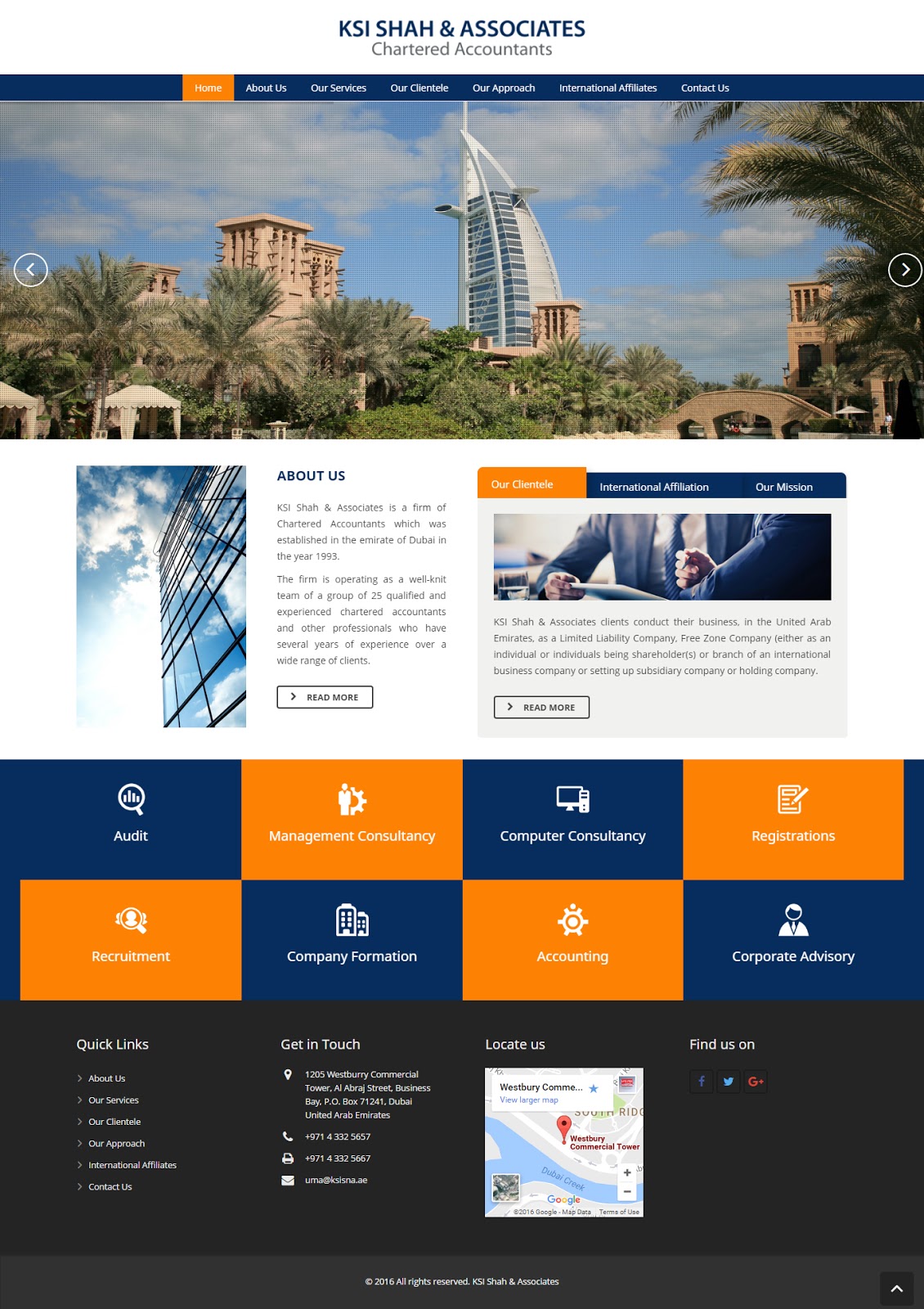Here’s the cleaned-up, detailed caption:

The image is a screenshot from the website of KSA Shaw and Associates. At the top center, "KSA Shaw and Associates" is prominently displayed in bold black letters, with "Chartered Accountants" written in gray beneath it. Below this, a black vertical rectangular bar divides the navigation menu. On the left, the "Home" button, highlighted in orange with the text in white, is followed by menu options including "About Us," "Our Services," "Our Choices," "Our Approach," "International Affiliates," and "Contact Us," all in white text.

Directly below the navigation menu, there are thumbnail images flanking a central image. On the left is a left-facing arrow button in white, and on the right, a right-facing arrow button in white. The central image features a half-moon-shaped building, with squared-off tan concrete buildings to the left and a backdrop of blue sky and white clouds. Trees and palm trees are visible to the right.

Moving further down, on the left side is a screenshot looking up the side of a building with reflective glass windows mirroring the sky. To the right of this, there is a section titled "About Us" with text that is too small to read, and a button at the bottom with a right-facing arrow that likely says "Read More."

Adjacent to this, there is a partially visible image of two men in blue suits. The man facing the camera wears a white shirt and blue tie, holding a tablet in his right hand, while the other man's back and partially visible right fist are shown.

At the top, a section highlighted in yellow features an hourglass icon followed by "International Affirmation" and "Our Mission." 

The bottom half of the page features a checkered yellow and blue background. On the left, there is a yellow button labeled "Audit," followed by "Management Consultancy," "Computer Consultancy," and "Registrations" in white text. Below this, starting with another yellow button, the options include "Recruitment," "Company Formation," "Accounting," and "Corporate Advisory," all in white text.